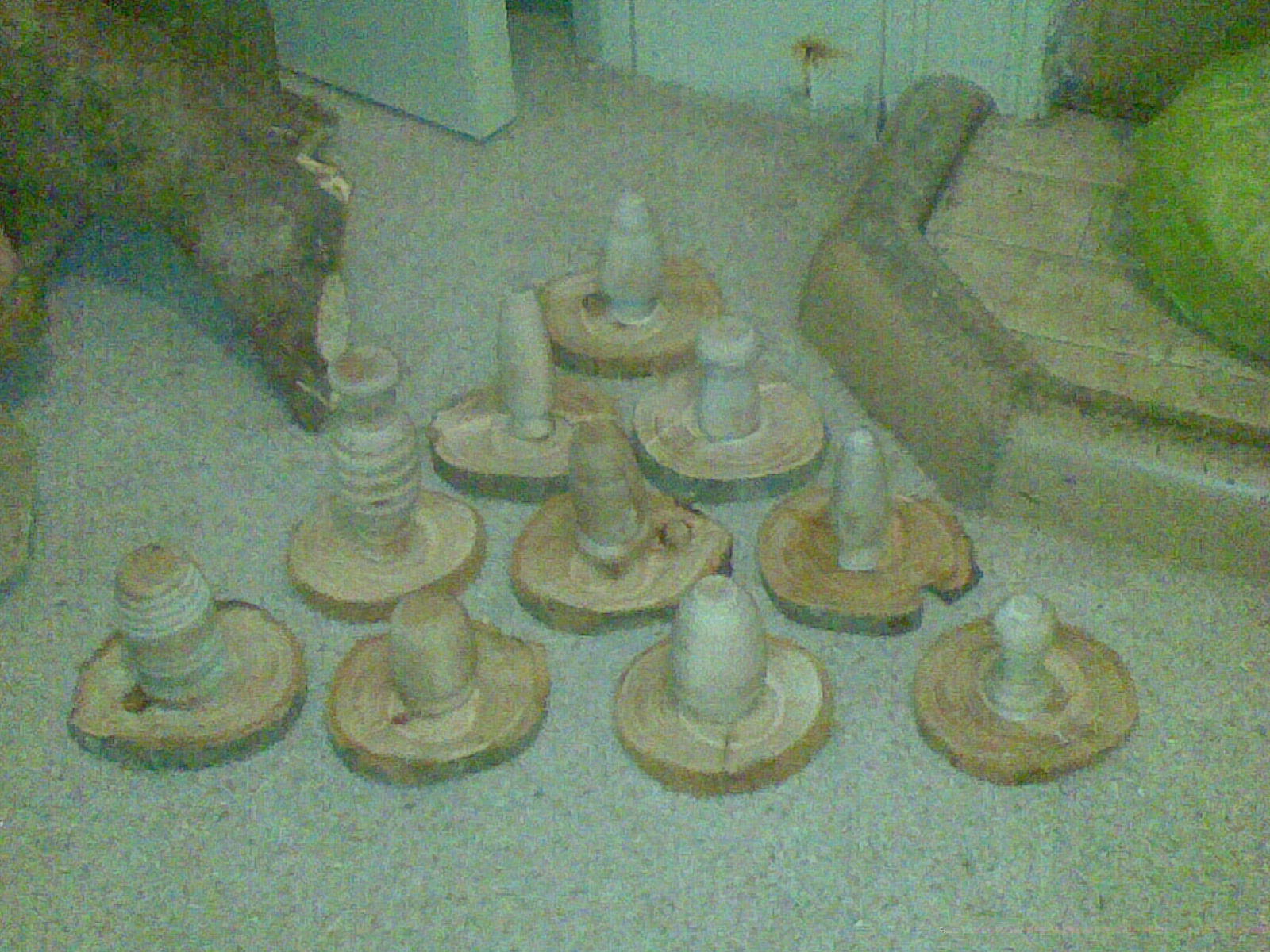The drawing illustrates an intricately arranged indoor display featuring a series of wooden stumps and carvings, each adorned with various ceramic pots and cylindrical objects of unique shapes and sizes. In the center, these wooden stumps are organized into a pyramid formation: four rows, with the number of stumps decreasing from four to one as they ascend, creating a triangular shape. Each stump, sliced from logs, serves as a pedestal for the ceramics resting atop, many of which appear to be upside down. A cow with black skin and a hint of white on its nose sniffs towards the bottom left, adding a whimsical touch to the scene. The backdrop includes a dark brown, driftwood-like tree drawing, set against a light tan background and complemented by white wall oiling with gray speckles. On the top right, there's a green bush providing a touch of nature, all laid out on a brick-tiled floor edged with a gray curb. Despite the graininess of the image, the detailed arrangement and variegated hues of the ceramics and wooden elements offer a captivating visual mosaic.